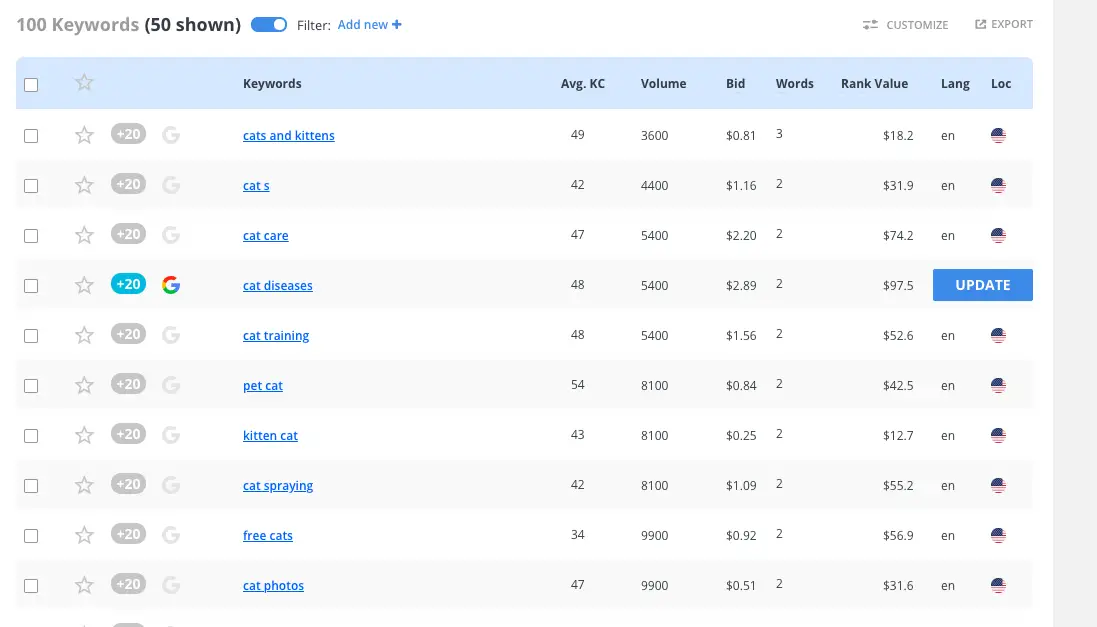The image depicts a detailed table used for keyword analysis. In the top left corner, it mentions "100 keywords (50 shown)," and in the upper right-hand corner, there are options for toggling a switch, filtering, adding new entries, customizing, and exporting data.

The table headers include the following categories: Keywords, Average KC, Volume, Bid, Words, Rank Value, Lang, and Lock. On the left side of the table, there are multiple rows with boxes; a column of stars follows this, where each row displays a "+20," except the fourth box down, which is highlighted in blue while the others remain gray.

Associated with the highlighted "+20" is a rainbow "G" in the subsequent column. The keyword rows, from top to bottom, are as follows: "cats and kittens," "cat ass," "cat care," "cat diseases," "cat training," "pet cat," "kitten cat," "cat spraying," "free cats," and "cat photos." Corresponding to these keywords, the "Average KC" values are 49, 42, 47, 48, 48, 54, 43, 42, 34, and 47, respectively.

For the "Volume" category, the values listed are 3,600, 4,400, 5,400, 5,400, 5,400, 8,100, 8,100, 8,100, 9,900, and 9,900. The "Bid" amounts are $0.81, $1.16, $2.20, $2.89, $1.56, $0.84, $0.25, $1.09, $0.92, and $0.51, respectively. In the "Words" column, the top entry is 3, while the rest are populated with the number 2.

For the "Language" category—and the "Location" represented by a picture of the US flag—all entries are marked English.